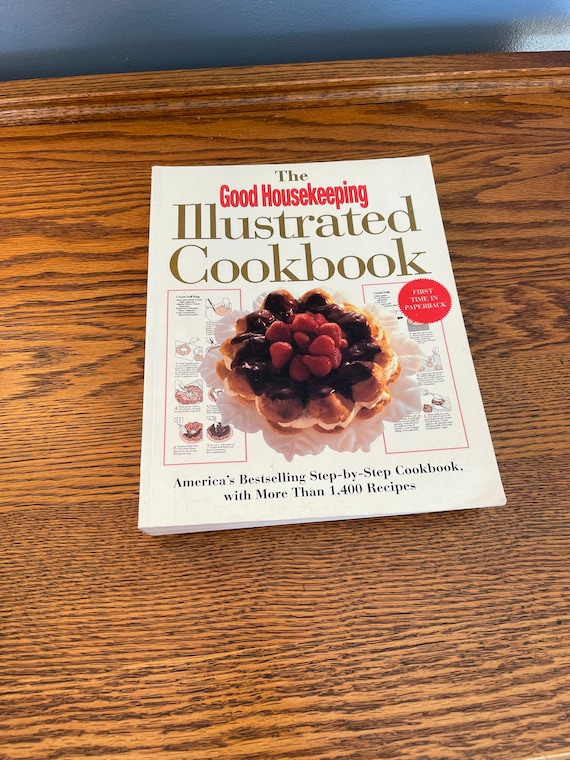This is a photo of a softcover, large edition of the Good Housekeeping Illustrated Cookbook, lying on a wood grain table. The cover features the title "Good Housekeeping" in red block letters, while "Illustrated Cookbook" is in gold block letters. A red ribbon declares "First Time in Paperback." Centered on the cover is an ornate, star-shaped dessert featuring a chocolate-topped cake with a dome of red raspberries on a white background. Flanking the dessert, there are two text boxes likely detailing recipe steps and book contents. Below the image, it states in black text, "America's Best-Selling Step-by-Step Cookbook with more than 1,400 recipes." The upper edge of the frame shows a glimpse of a blue-gray wall.